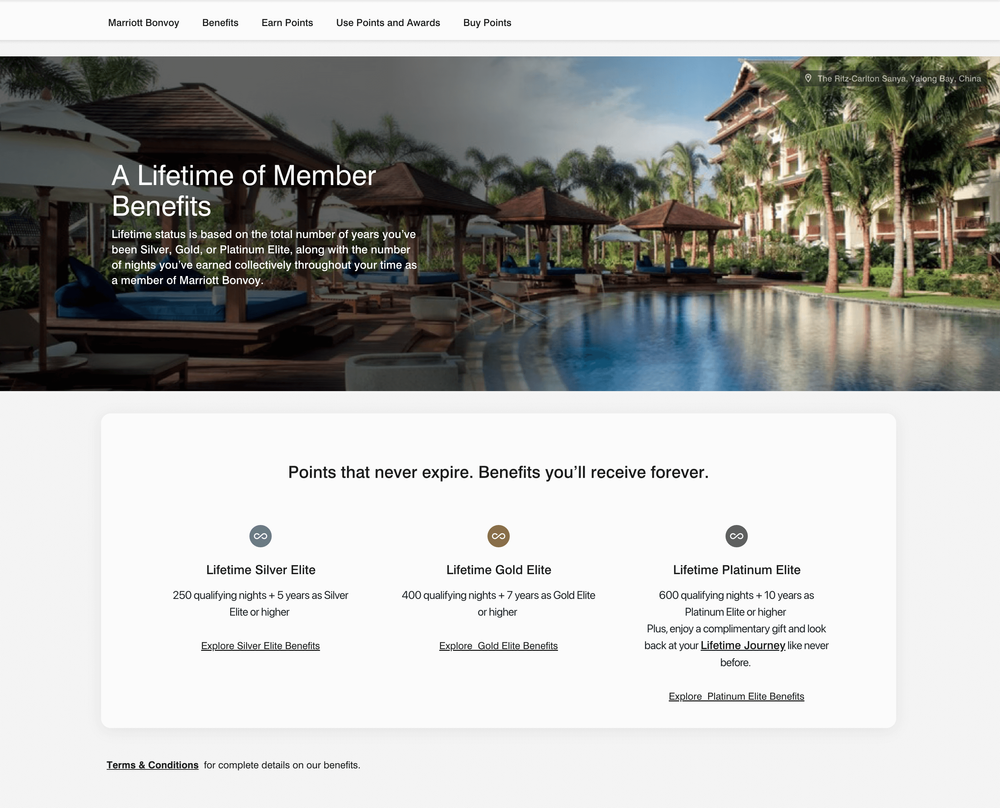**Caption: Detailed Overview of Marriott Bonvoy Lifetime Member Benefits and Images of The Ritz-Carlton, Sanya, Yalong Bay, China**

In this informative visual, the left side highlights various Marriott Bonvoy member benefits such as "Earned Points," "Used Points and Awards," and "Buy Points." Adjacent to this information, it showcases the impressive facilities at The Ritz-Carlton in Sanya, Yalong Bay, China. A stunning image features a luxurious pool surrounded by lush trees and greenery. To the right of the pool, there are inviting lounge areas equipped with comfortable beds and canopies, all framed by elegant wooden accents.

The visual also elaborates on the prestigious Marriott Bonvoy Lifetime Member Benefits. It explains that achieving lifetime status depends on the total number of years a member has held Silver, Gold, and Platinum status, as well as the number of qualifying nights. Key milestones for Lifetime Membership include:

1. **Silver Lifetime Status**: Achieved with 250 qualifying nights and 5 years as Silver Elite or higher. Members enjoy Silver Elite Benefits.
2. **Gold Lifetime Status**: Achieved with 400 qualifying nights and 7 years as Gold Elite or higher. Members can explore Gold Elite Benefits.
3. **Platinum Lifetime Status**: Achieved with 600 qualifying nights and 10 years as Platinum Elite or higher. Members enjoy Platinum Elite Benefits and a complimentary gift.

Additionally, it emphasizes that points never expire and benefits last forever. Explore detailed terms and conditions to understand all the privileges associated with these elite statuses.